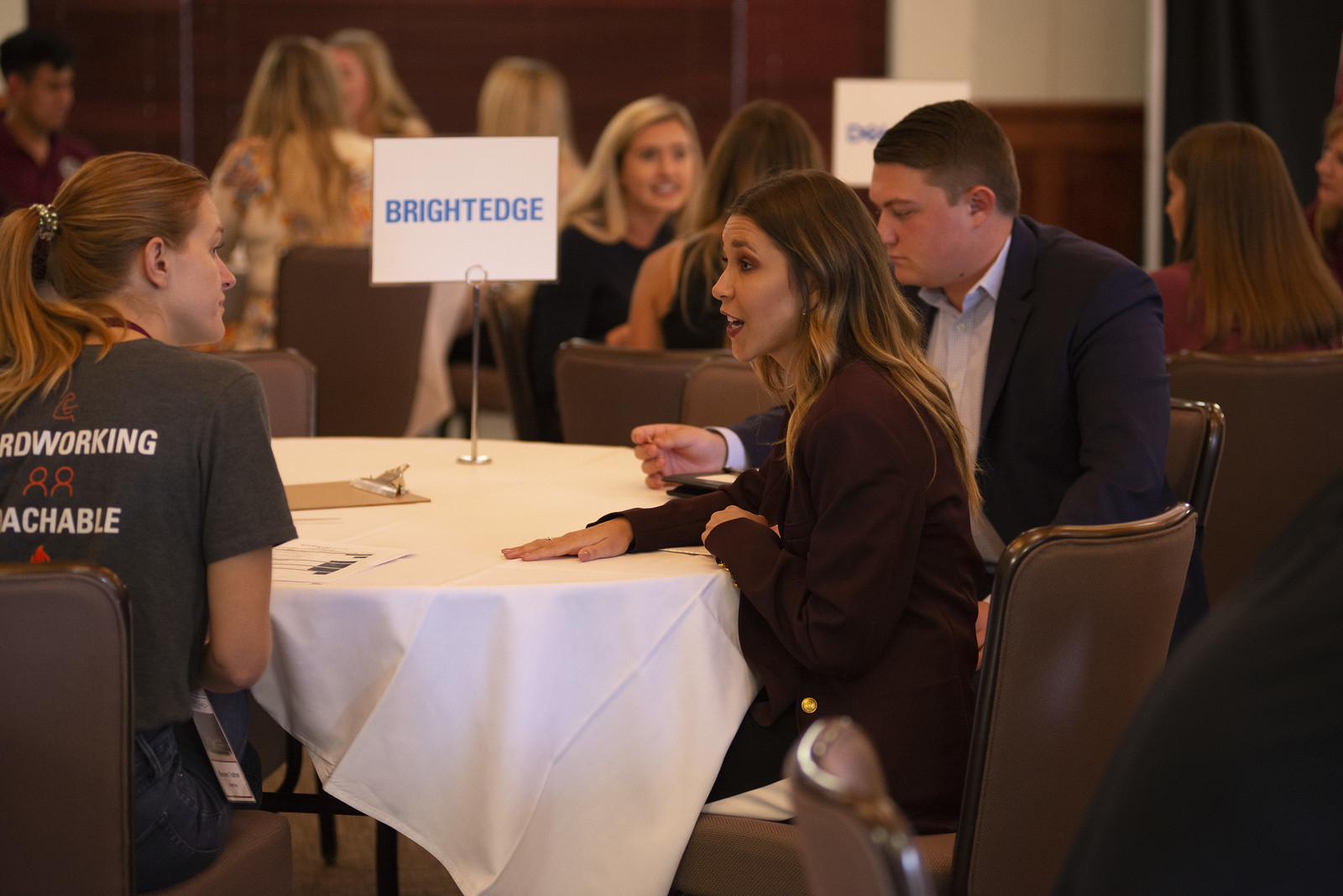The photograph depicts a busy banquet room filled with several tables and young individuals engaged in conversation. In the foreground, a prominent table with a white tablecloth is the focal point. Seated at this table, a girl on the left wears a t-shirt with her hair tied in a ponytail, and she is conversing with a woman directly across from her, who has long brown hair and is clad in a burgundy shirt. According to another observation, the woman could be wearing a black sport coat or sweater instead. Next to her, a young man, donned in a blue suit coat over a white dress shirt, listens silently. On this same table, there is a visible sign that reads "Brightedge" in blue letters. Surrounding this main scene, several other tables filled with youthful men and women can be seen, though details are more obscured in the background. Distributed around the tables are brown chairs, reinforcing the cohesive setup of the banquet room. Other tables also appear to have signs, but they are partially blocked and illegible due to the positioning of the people.